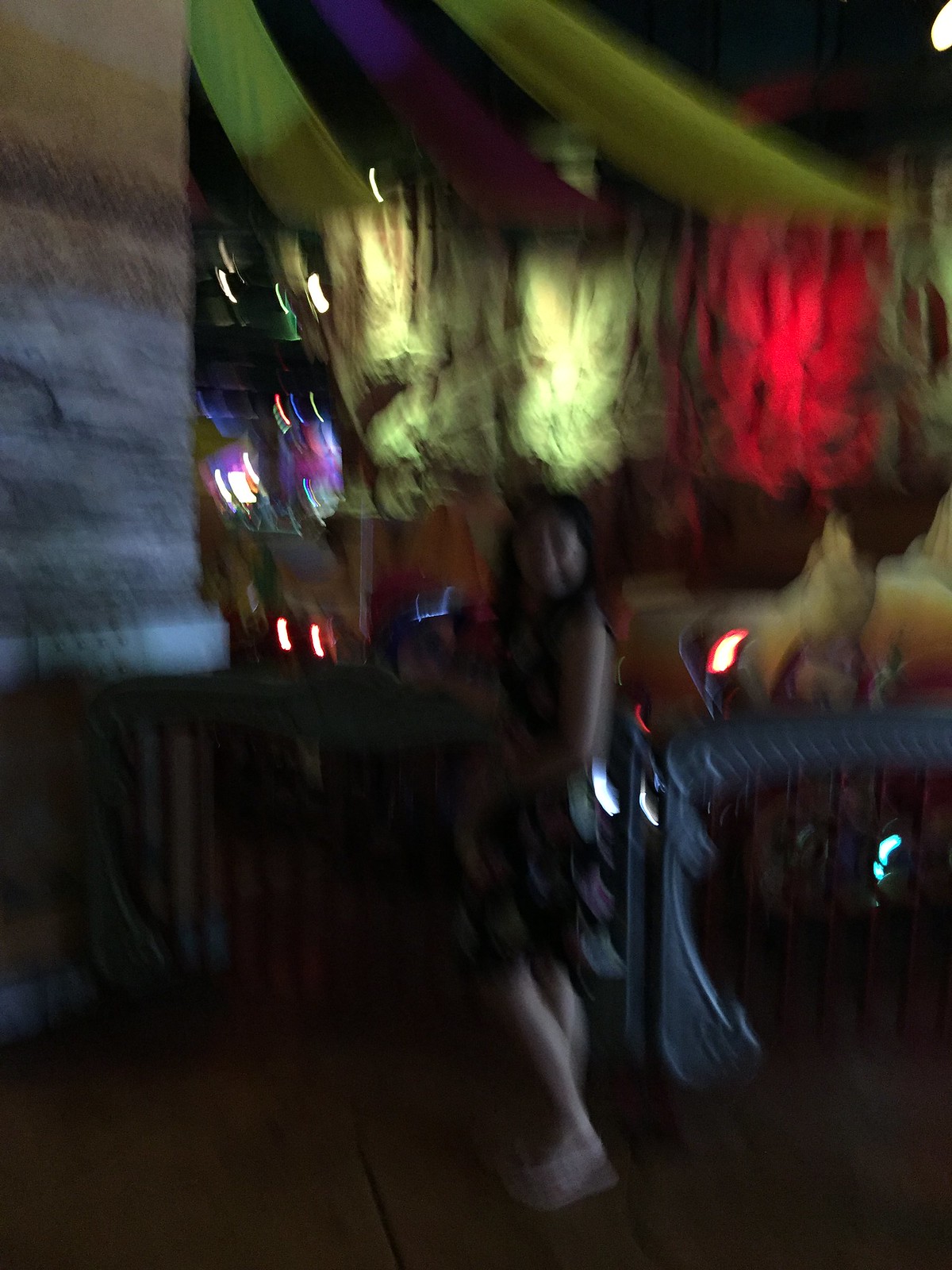The photograph captures a dimly-lit scene, likely at night, featuring a woman standing next to a round table in what appears to be a nightclub or bar, though the exact setting is ambiguous. She is dressed in a black sleeveless or short-sleeved dress and cream-colored sandals with straps across the top, possibly wedges. Her medium-length curly hair, which is either brown or black, cascades around her shoulders as she faces the camera, seemingly smiling, though the image is blurred.

She stands next to a black wrought iron railing that curves into an arched balcony area, suggesting an upper level overlooking another part of the venue. The background features walls of exposed brick and possibly stone, adorned with various colorful, illuminated hangings—one in green, one in red, and another perhaps in cream. These hangings might be pieces of art or fabric, contributing to the eclectic decor. Additional pale green swatches of fabric are seen hanging overhead, connected to the wall. The ambiance is further accentuated by blurry neon lights in the far background, which could belong to the bar or slot machines, hinting at the lively, vibrant atmosphere of the scene.